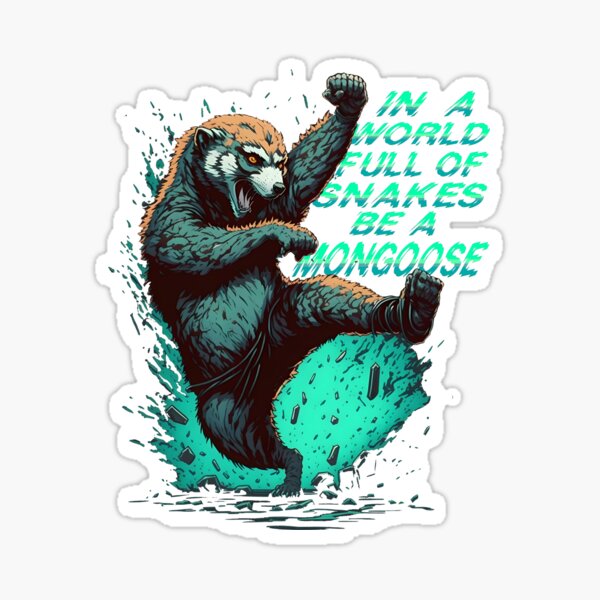This image features a dynamic sticker of an animated mongoose performing a spirited karate move. The mongoose is depicted standing on one foot, with the other leg kicking up high. Its left arm is extended upwards, and its right arm is positioned near its midsection in a fierce fighting stance. The mongoose, with animated, fierce red eyes and an open mouth, appears to be in motion, as though it is shouting "hi-yah." It has tan fur on its legs and arms and extra hair on its head that is also tan.

The background of the sticker is white, adorned with splatters of green and teal, giving an impression of an explosive burst behind the mongoose. The sticker has a jagged, scalpel-cut edge that follows the outline of the mongoose and the surrounding chaotic elements. Alongside the animated figure, the inspirational text "In a world full of snakes, be a mongoose" is presented in contrasting ombre green lettering, adding a motivational touch to the image. The mongoose appears to be breaking through a wall, emphasizing its powerful and fearless demeanor. Overall, the sticker captures a sense of action and defiance with its vibrant colors and energetic composition.